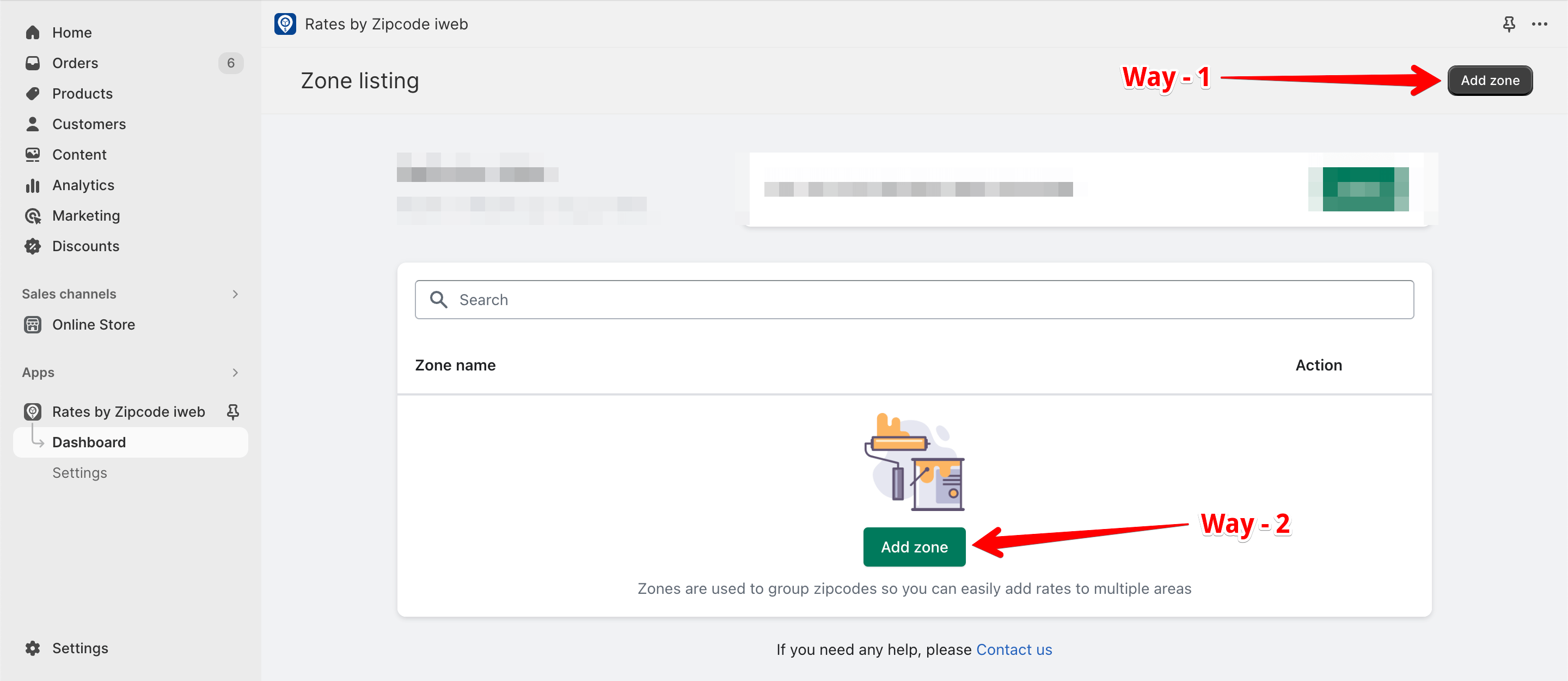The image is a screenshot from a website featuring a "Zone Listing" page. In the upper right-hand corner, a red arrow has been digitally added, pointing to the right towards a button labeled "Add Zone." Next to the arrow, the text "way-1" is displayed in red. On the bottom right-hand side, another red arrow points to the left towards a similar "Add Zone" button, accompanied by the text "way-2."

In the top left corner of the page, there is a vertical sidebar menu with various options, each accompanied by an icon. The first option has a house icon and is labeled "Home." Below it, a rectangle icon is paired with the label "Orders." Following this, a price tag icon indicates "Products," and a silhouette icon represents "Customers." Additional options include "Content," "Analytics," "Marketing," and "Discounts," each with their respective icons. Further down the sidebar, the "Sales Channel" section lists "Online Store" and "Rates by Zip Code," with "Dashboard" appearing at the end of this section.